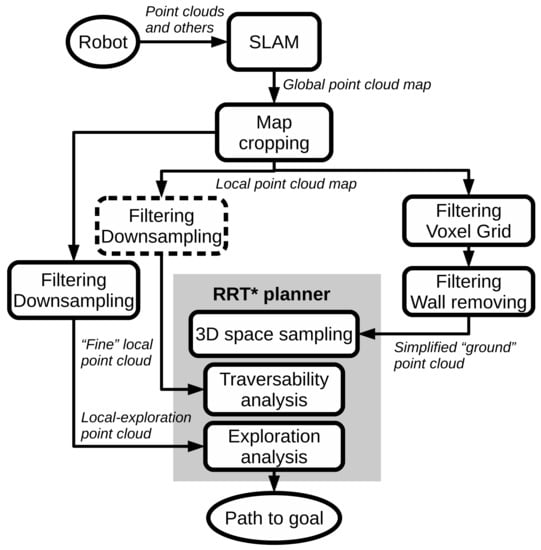The black-and-white diagram illustrates a detailed workflow, starting from a robot inside an oval shape located in the upper left corner. Adjacent to it, a right-pointing arrow indicates the progression to a rectangle labeled "SLAM." Above this arrow, annotations mention "point clouds" and other points. From "SLAM," a downward arrow leads to a rectangle containing the words "global point cloud map." 

Additionally, another arrow progresses downward to a rectangle labeled "map cropping." To the left of this, a horizontal line with an attached downward arrow points toward another series of rectangles that represent various filtering processes, including filtering down sampling, voxel grid, and wall removing. These interconnected elements further lead to "3D space" and "traversability analysis."

The workflow continues with arrows pointing to "exploration analysis" and finally concludes with "path to goal." In the bottom center of the diagram, a light gray box contains several of these rectangles and is labeled "RRT* planner."